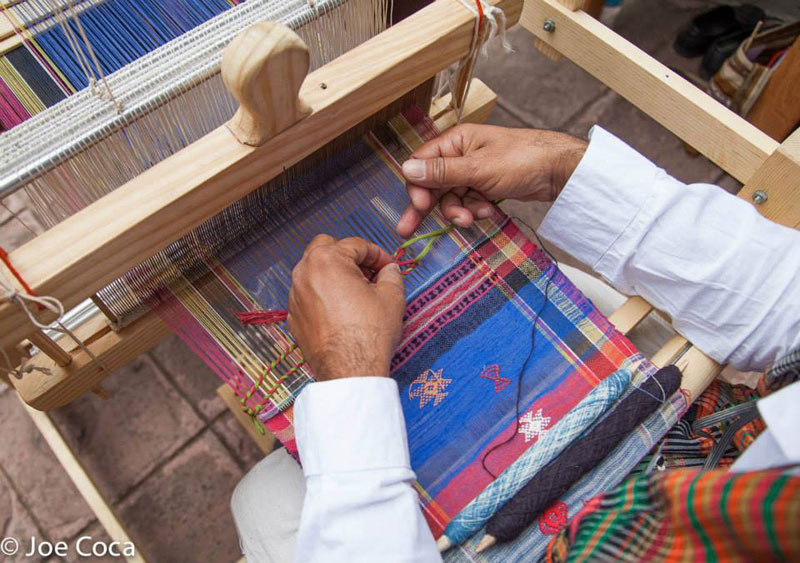The image captures a close-up of a man's hands actively weaving on a wooden loom, which appears to be made of pine. His hands, emerging from long white sleeves, are threading various colored yarns—black, blue, orange, red, white, and pink—into an intricate fabric. The fabric features detailed patterns, including a red hourglass on a blue background and a snowflake-like symbol. Below the loom, several spools of thread are visible. The well-worn brown cobblestone floor beneath adds to the historical and artisanal ambiance of the scene. In the bottom right corner, the text 'copyright Joe Coca' is noted.